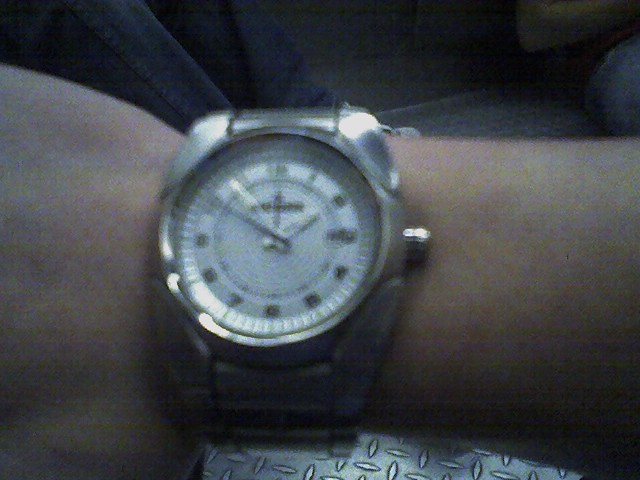This image showcases an elegant wristwatch with a polished chrome body and a matching metal band. The watch face is white, adorned with numerals presumably written in Arabic script, marking the hours from 1 to 12. It features three hands: an hour hand, a minute hand, and a second hand. The time displayed on the watch is approximately 12:10 and 54 seconds. The sleek and sophisticated design highlights the watch's refined craftsmanship and attention to detail.